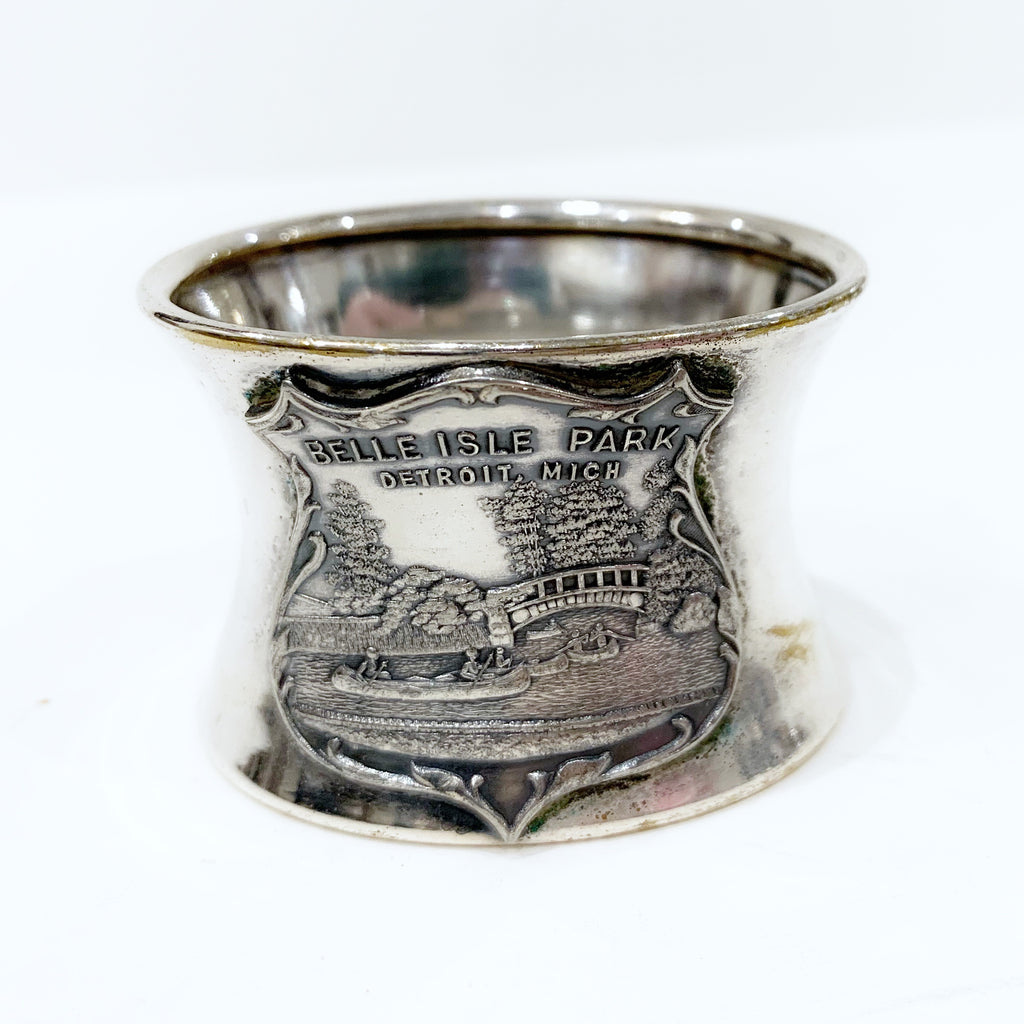This photograph showcases a close-up of a small, tarnished silver shot glass or possibly a spittoon, set against a white background. The item, which appears quite old, features an engraved badge-like emblem on its front, reading "Belle Isle Park, Detroit, Michigan." Below the inscription, the engraving depicts a scenic view of Belle Isle Park, complete with trees, a quaint bridge, a body of water, and people canoeing. The silver item has a wide-lipped base that narrows in the middle before expanding again at the bottom, giving it a distinct, somewhat rustic appearance. The intricate details and the tarnishing suggest that it might be a vintage souvenir, potentially from the 1930s or 40s.